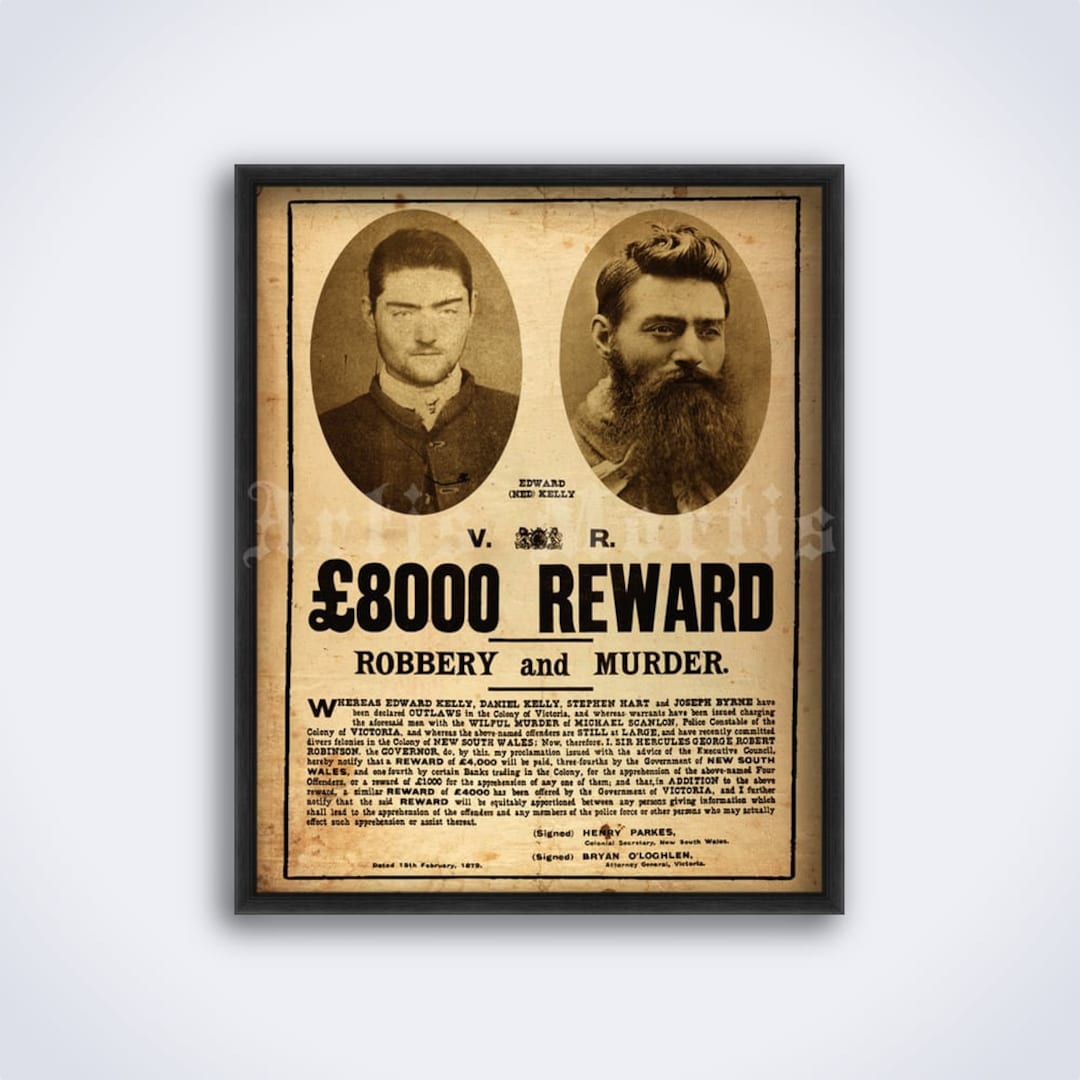The image depicts a vintage-style wanted poster, likely from England due to the mention of an 8,000-pound reward. The poster, framed in black, is set against a bright white background and features a tan sheet of paper with a black border. At the top, two oval-shaped sepia-toned photographs present one man clean-shaven on the left, and another with a long beard and longer hair on the right. Both men are slightly angled to the right and dressed in period clothing reminiscent of theme park costumes. Above the reward amount, the barely legible text begins with the letter "R," likely serving as a watermark, with "A-R-T-I-S M-A-R-T-I-S" discernible in the center of the image. Prominent, bold text reads "£8,000 reward," followed by "robbery and murder." Despite much of the accompanying text being too small or blurred to read clearly, names like Edward Kelly and Joseph Byrne can be distinguished. The detailed nuances of attire, text, and the poster's aged appearance lend an authentic, historic ambiance to the photograph.